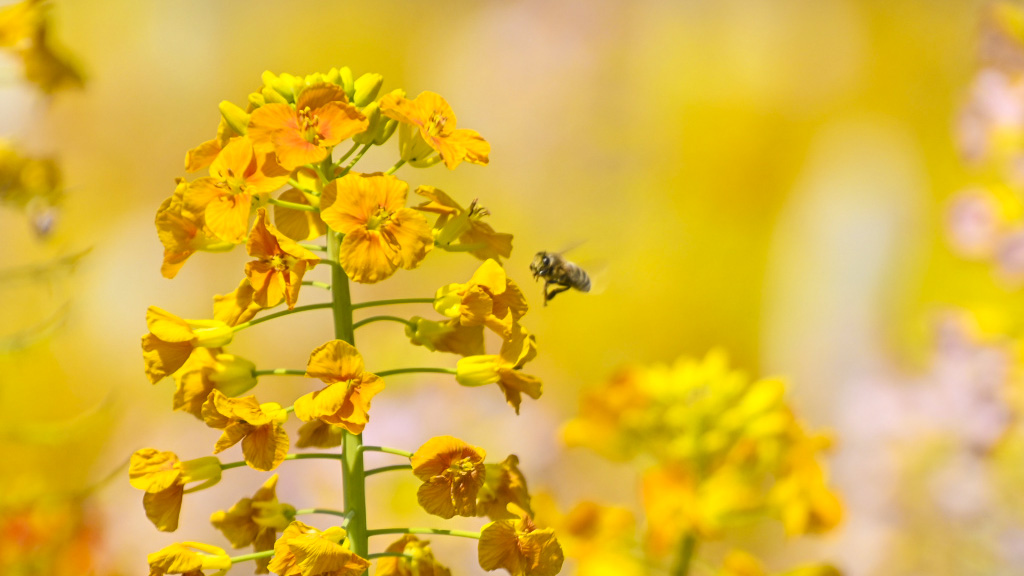The image is a close-up of a vibrant green stem with multiple branches, each adorned with bright yellow flower buds. A bee, black and yellow with fuzzy details, is captured mid-flight on the right side of the frame, almost at the center, its wings blurred in motion. The background is artistically out of focus, revealing a vast field dominated by yellow hues, suggesting more of the same plant, and possibly a hint of pink flowers. The overall impression is a vivid and professional portrayal of nature, emphasizing the beauty and activity in this bustling outdoor scene.